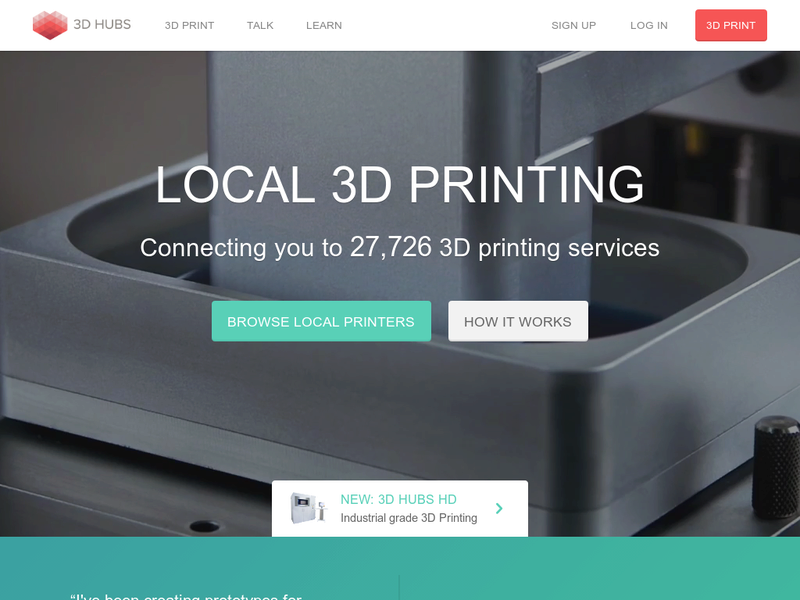The top portion of the background features a design with white and red elements. On the left side, several red triangles come together to form a bulky heart shape. To the right of this heart shape, the text "3D Hubs" appears in black. Adjacent to the text are links in black that say "3D Print," "Talk," "Learn," "Sign up," and "Log in." Below these, there's a red rectangle with the text "3D Print" in white.

In the background, the image appears to show a piece of 3D printing equipment, although it is zoomed in so closely that the entire machine isn't visible. You can see a silver base with some spacing and another piece of metal in the center, but the full apparatus remains out of view.

Overlaying this background in white, capitalized text are the words "LOCAL 3D PRINTING." Below this, in white text with only the first letter capitalized, it reads "Connecting you to 27,726 3D printing services."

There are two call-to-action rectangles underneath this text. The first rectangle is a sea breeze green color with white, capitalized text that says "BROWSE LOCAL PRINTERS." The second rectangle is an off-white color with gray, capitalized text that says "HOW THIS WORKS."

At the bottom of the image, an off-white rectangle contains a message in sea breeze green, capitalized text saying "NEW 3D HUBS HD." Below this, in gray text with only the first letter and the 'D' in 3D capitalized, it says "Industrial grade 3D printing."